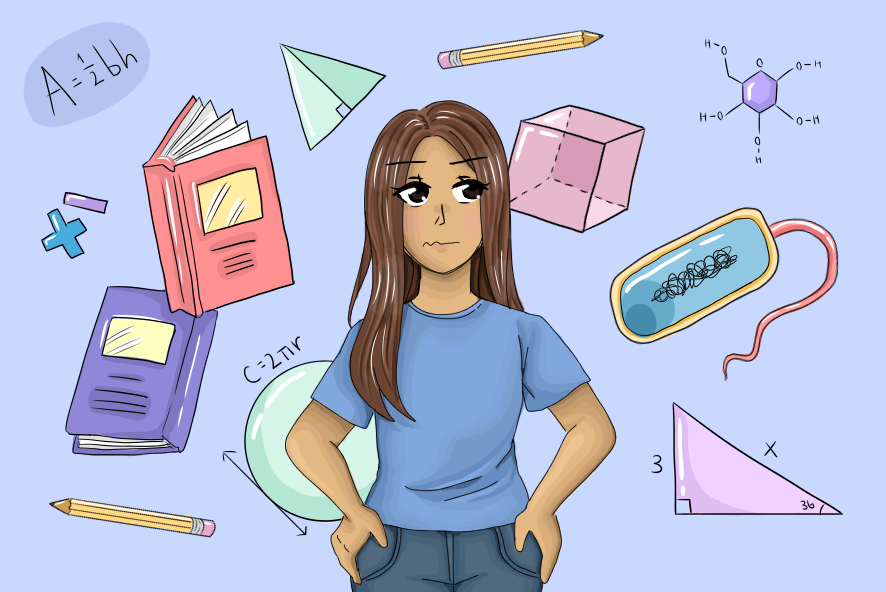This illustration depicts a cartoon girl from the waist up, rendered in an anime-influenced art style. She wears blue jeans and a light blue, short-sleeve t-shirt, with her long brown hair cascading past her armpits, partially brushed to one side. Her large brown eyes exhibit a confused expression, glancing up and to the right, with a scribble-shaped mouth conveying discomfort. Surrounding her are numerous colorful, science and math-related drawings floating in a light blue background. To her left, there's a yellow pencil, a purple textbook above an orange one, and a plus and minus sign. Further up is a dark blue oval labeled "A = 1/2 BH." On her right side, there's a green triangle and another yellow pencil. Adjacent is a pink cube and the chemical formula "H-O-H-O-O-O-H-O-H-O-H." Additional elements include drawings of various geometric shapes, math equations, and possibly biological items, suggesting her anxiety or confusion about these academic subjects.